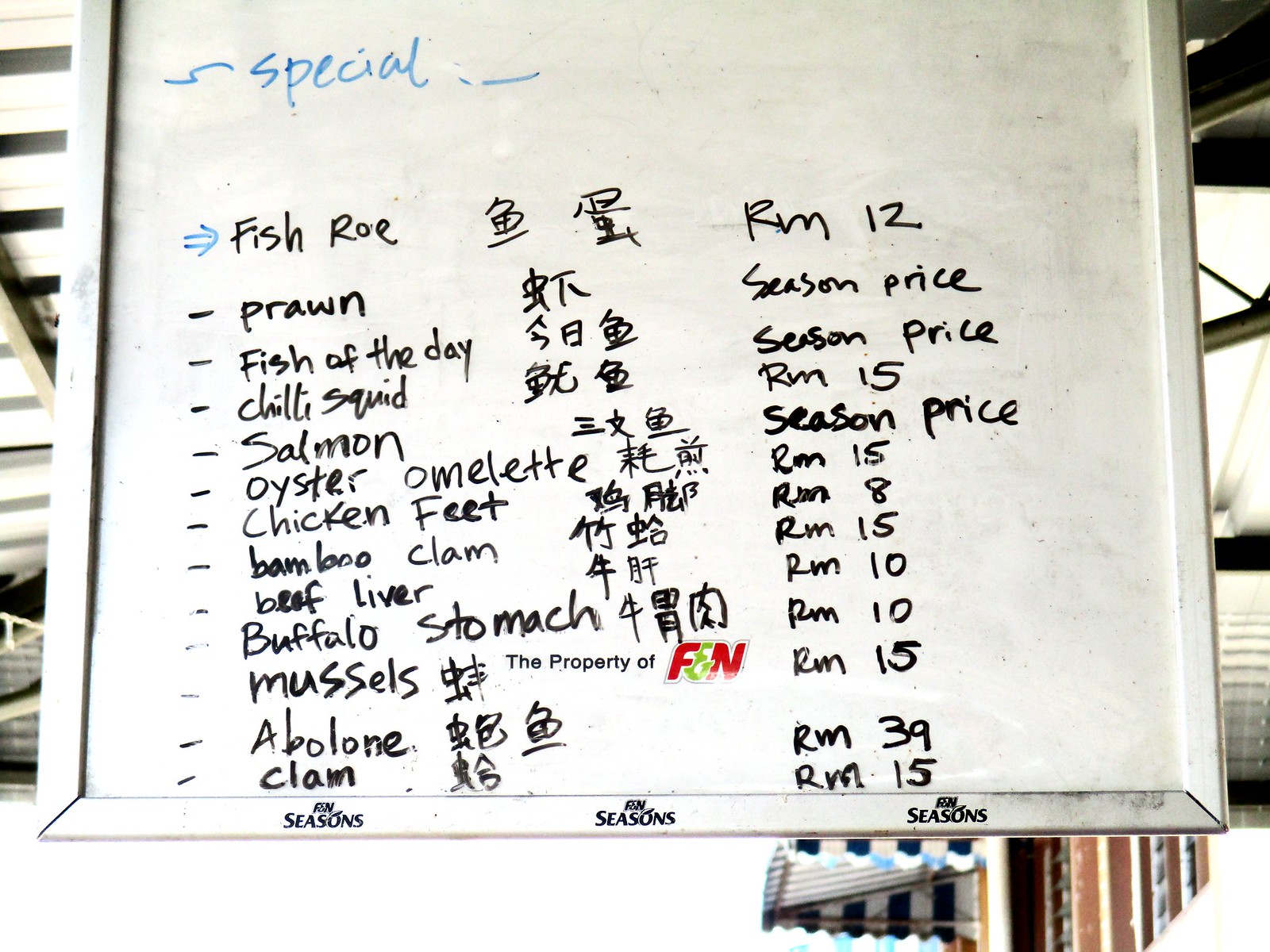This horizontal rectangular image shows a slightly worn and messy whiteboard, which appears to be hanging from the ceiling, against a backdrop featuring a metal roof on the left. The whiteboard serves as a menu in what seems to be a butcher or fish shop. Displayed prominently in blue text at the top left is the word "Special" with a blue arrow next to it. The rest of the text is predominantly in black, listing various items such as fish roe, prawns, salmon, mussels, buffalo stomach, and chili squid, among others. Each item is written in English and is accompanied by Chinese characters next to it. The board specifies the location or pricing for each item, with several items listed as "season price" and others directing customers to specific rooms, like "Room 12," "Room 10," and "Room 15," indicating where the items can be found. Notably, the bottom of the whiteboard displays the words "F and N seasons" and the logo, which states "The property of F and N," with the letters "F" and "N" in red and the ampersand in green.